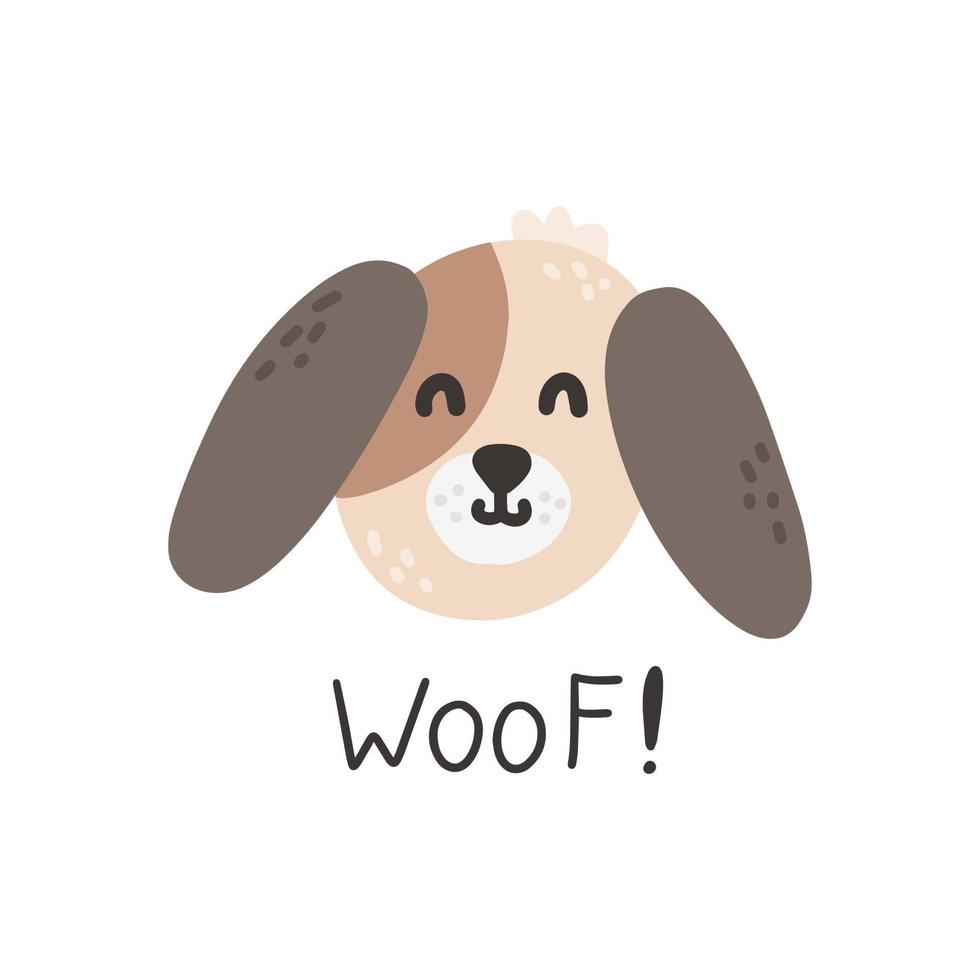This image features a playful, simplistic, and childlike cartoon illustration of a dog's head set against a white background. The dog's head is round and beige, adorned with a tuft of tan hair. It features thick-lined, upside-down U-shaped eyes and a small black nose, characterized by a triangular shape. The muzzle is white, with two small curved lines for the mouth, resembling upturned U's. A distinctive dark brown patch covers one eye, adding a touch of character. The ears are elongated ovals, taupe in color, that look as if they are just lightly attached to the head. Underneath the dog’s head, in a handwriting-styled font with relatively thin linework, the word "WOOF!" is inscribed. Notably, the exclamation point is quite thick compared to the rest of the text, drawing immediate attention. The overall format is square, with no additional elements, shadows, or background, giving the illustration a floating appearance.